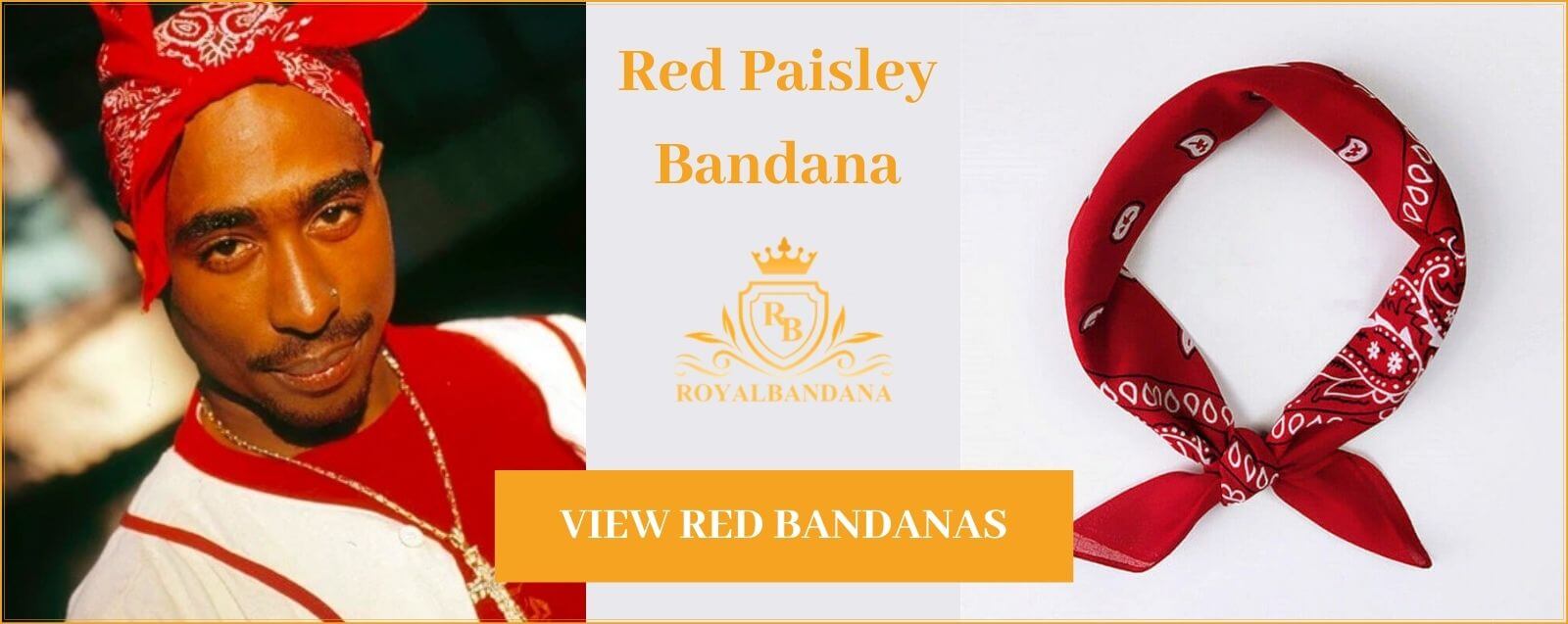The image features a yellow-outlined rectangular layout. On the left is a photograph of an African-American man with a mustache, black goatee, and a nose piercing. He has brown eyes, black eyebrows, and wears a red bandana tied at the top of his forehead. His attire includes a red and white shirt with a large cross symbol, accompanied by a gold necklace that also has a cross pendant. The background behind him is blurred with black and white tones. 

In the center of the image, an orange rectangle displays the text "View Red Bandanas" in yellow. To its right, on a white background, appears the phrase "Red Paisley Bandana" in yellow font. Below this text is a logo featuring a crown above a shield with the letters "RB" and decorative leaves, labeled "Royal Bandana."

On the far right side, another red bandana is shown tied into a circular knot, set against a completely white background. The entire composition is bordered by a yellow frame.